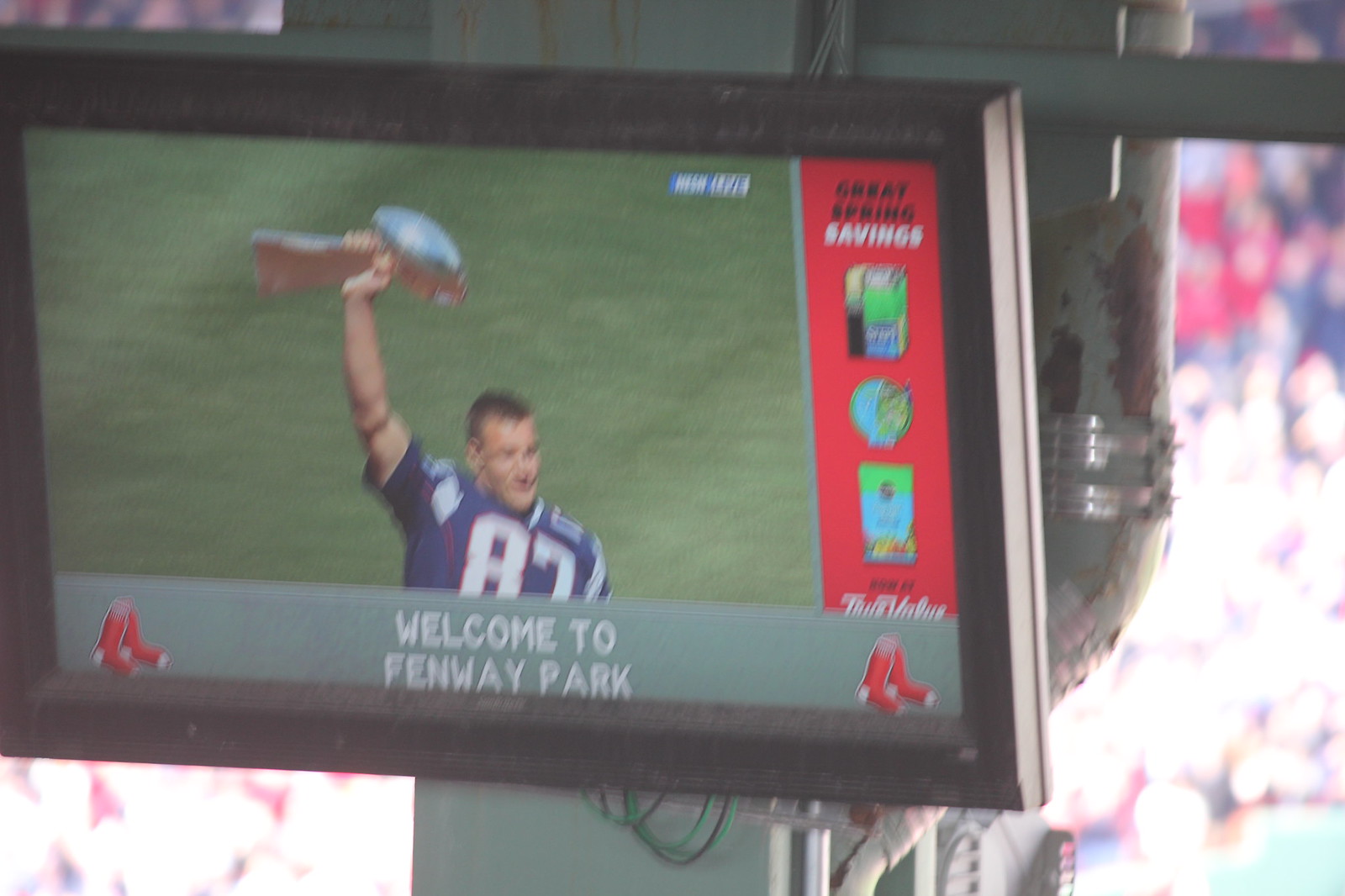This is a detailed photograph of a small, rectangular TV screen with a black border, mounted on a metal post within a room. The TV displays a sports image, featuring a man in a blue football jersey with white letters, holding a silver football trophy aloft. The screen banner reads "Welcome to Fenway Park" in white letters, and there's a Red Sox insignia, adding a layer of confusion between football and baseball imagery. Below the banner, the number 87 is visible on the man's jersey. Behind the TV, there is a light green horizontal board and a dark green, rusted pipe with an aluminum clasp, accompanied by another horizontally running pipe. The background includes blurry sections of red and white colors, suggesting a busy and multi-colored interior, possibly in a bar or restaurant setting, with some adverts reading "Great Spring Savings" and images of household items. The scene is further framed by nearby windows, contributing to the complex and layered visual composition.